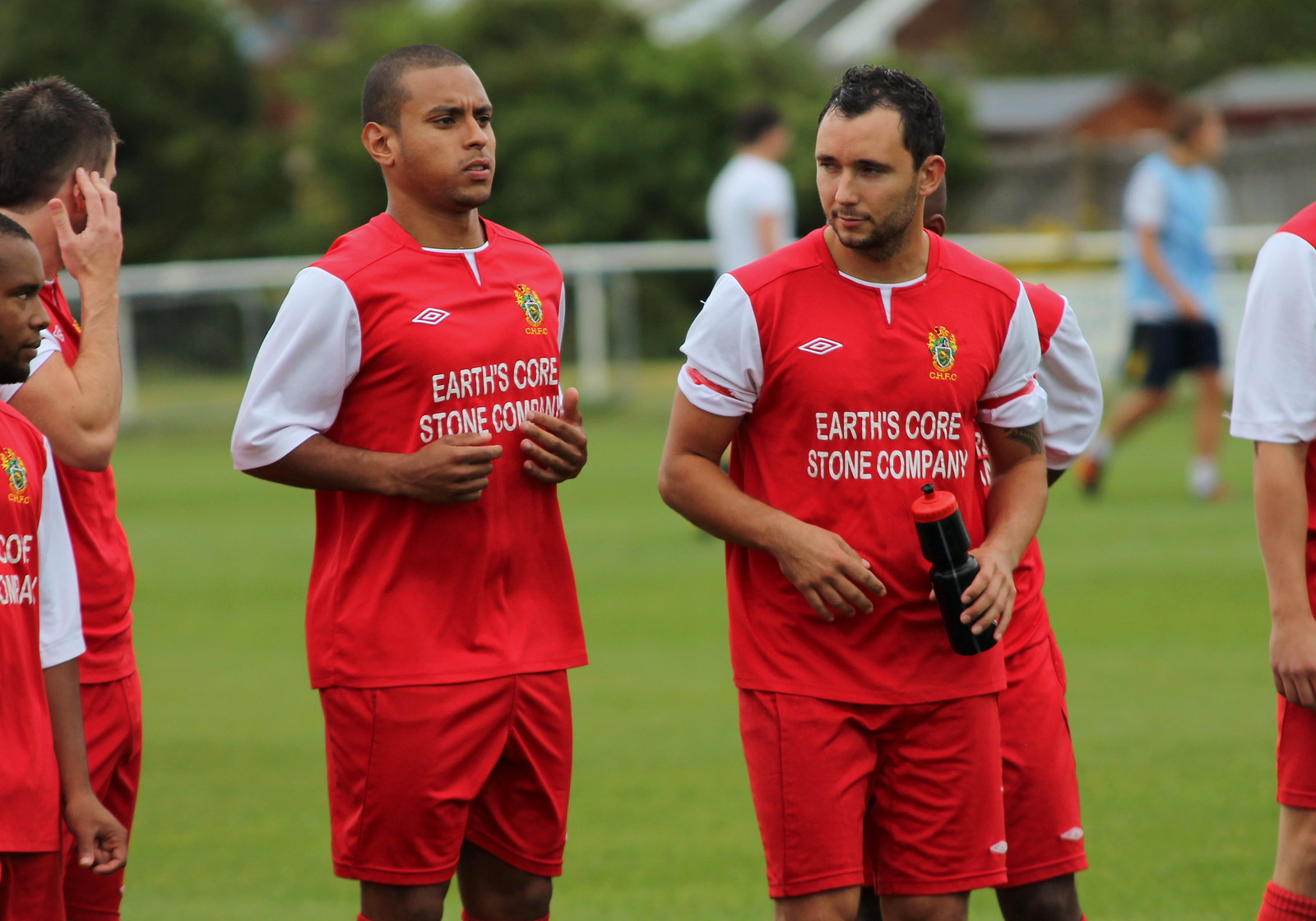This photograph appears to capture a group of men at what seems to be a sporting event, most likely soccer, given their athletic attire and the green grass they are standing on. The men in the foreground are prominently displayed, wearing matching red jerseys with white sleeves and red shorts. The jerseys are emblazoned with "Earth's Core Stone Company" and feature small logos on both the upper right and upper left sides of the chest. The man in the front right of the image holds a black and red water bottle in his left hand. 

In the background, the scene is slightly blurry but discernible. You can see a low white fence and some green shrubs. There are other men behind the main subjects, one in a white shirt and another in a light blue shirt with black shorts, suggesting they may be part of a different team or the event's audience. There are also vague outlines of what could be trees and possibly a building further back. The overall atmosphere suggests that these men are either preparing for, or taking a break from, a game, with one man appearing to have his hand over his ear, perhaps listening to instructions or communicating with others.